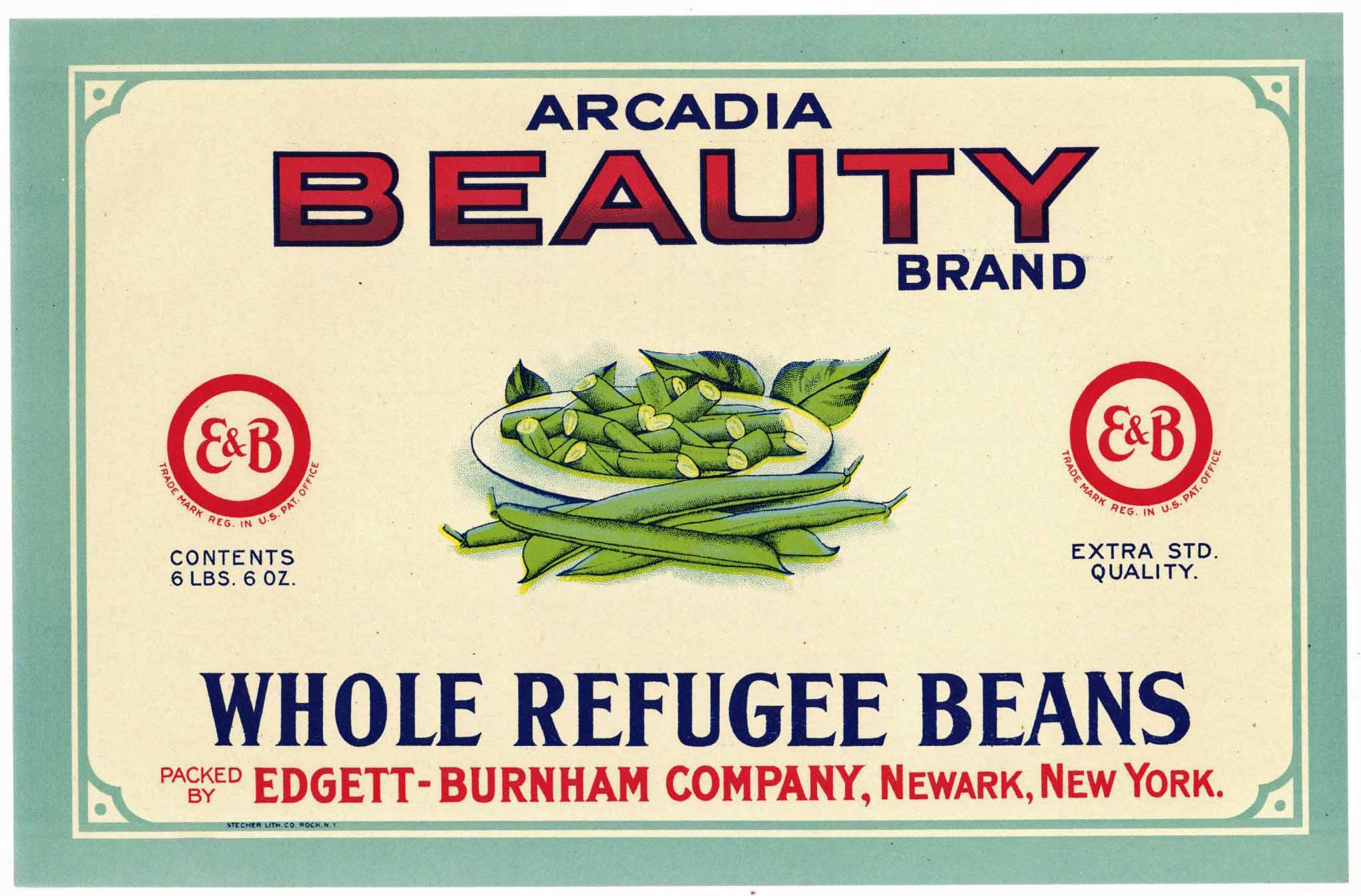The image appears to be an old-fashioned label, primarily in green and tan colors, with detailed text and graphics. At the top, "Arcadia" is prominently displayed, with "Beauty" in red letters below it, followed by "Brand" in black. Centered on the label, there's an illustration of a white plate with green beans—some of them whole and others snapped. To both the left and right of this, there's a red circle enclosing the letters "E&B." On the left side, beneath the circle, it reads "Content, 6 lbs, 6 oz," and on the right side, it states "Extra Standard Quality." Below the plate, the text "Whole Refugee Beans" is noted in blue, followed by "Packed by Etage Burnham Company, Newark, New York" in red at the bottom. The label’s vintage style suggests it might be from a company that is no longer in business.